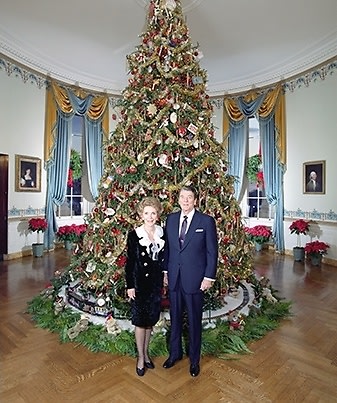In this image, President Ronald Reagan and First Lady Nancy Reagan are standing in an elaborately decorated room of the White House during Christmastime. The President, positioned on the right, is wearing a dark blue suit, white shirt, and a blue tie. Mrs. Reagan, on the left, is adorned in a stylish black dress with a white ruffled collar, complemented by black pantyhose and black shoes. They are in front of a towering Christmas tree that stretches up to the ceiling, its base encircled by a quaint train track and lush greenery. The room's herringbone-patterned hardwood floor frames the setting elegantly. Surrounding the Christmas tree, vibrant poinsettias in pots add to the festive atmosphere. Two windows, each draped with pale blue and gold curtains pulled back neatly, feature holly wreaths hanging midway down. The room, with its white curved walls and crown molding, gives an opulent backdrop, enriched further by the presence of framed photographs, although their subjects are indistinct.